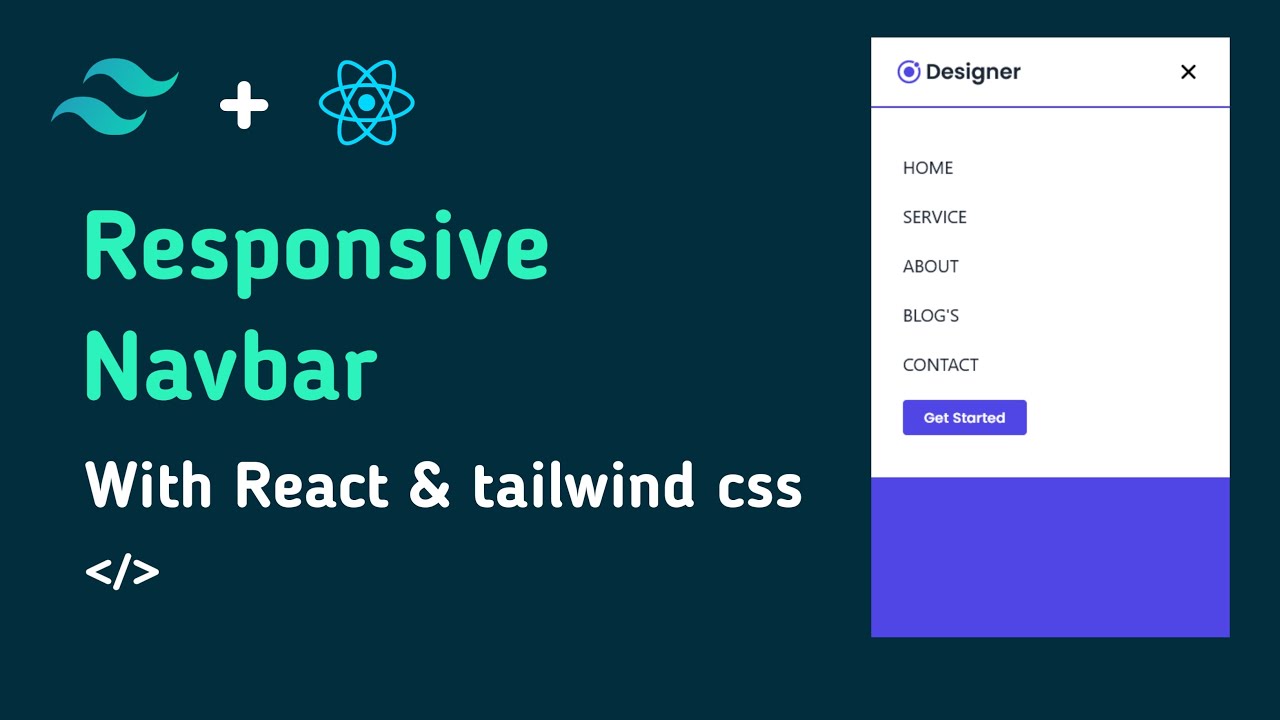The photographic image depicts a web page dominated by a navy blue color scheme. At the top of the page, two light blue, squiggly lines evoke the appearance of waves. Positioned nearby is a white plus sign and an intricate, circular pattern rendered in shades of blue, reminiscent of a physics graphic.

On the right side of the image, a white section stands out. This section features the word "Designer" in black font, accompanied by a blue circle. Near this area is an 'X' symbol and several navigation buttons labeled "Home," "Service," "About," "Blogs," "Contact," and "Get Started." Notably, the "Get Started" button is displayed in white font against a blue button.

Towards the bottom of the page, a lighter blue banner captures attention with the text "Responsive Nav Bar" in a large, green font. Just beneath it, the phrase "With React and Tailwind CSS" appears in a smaller, white font. The lower section of the page is adorned with several additional graphics.